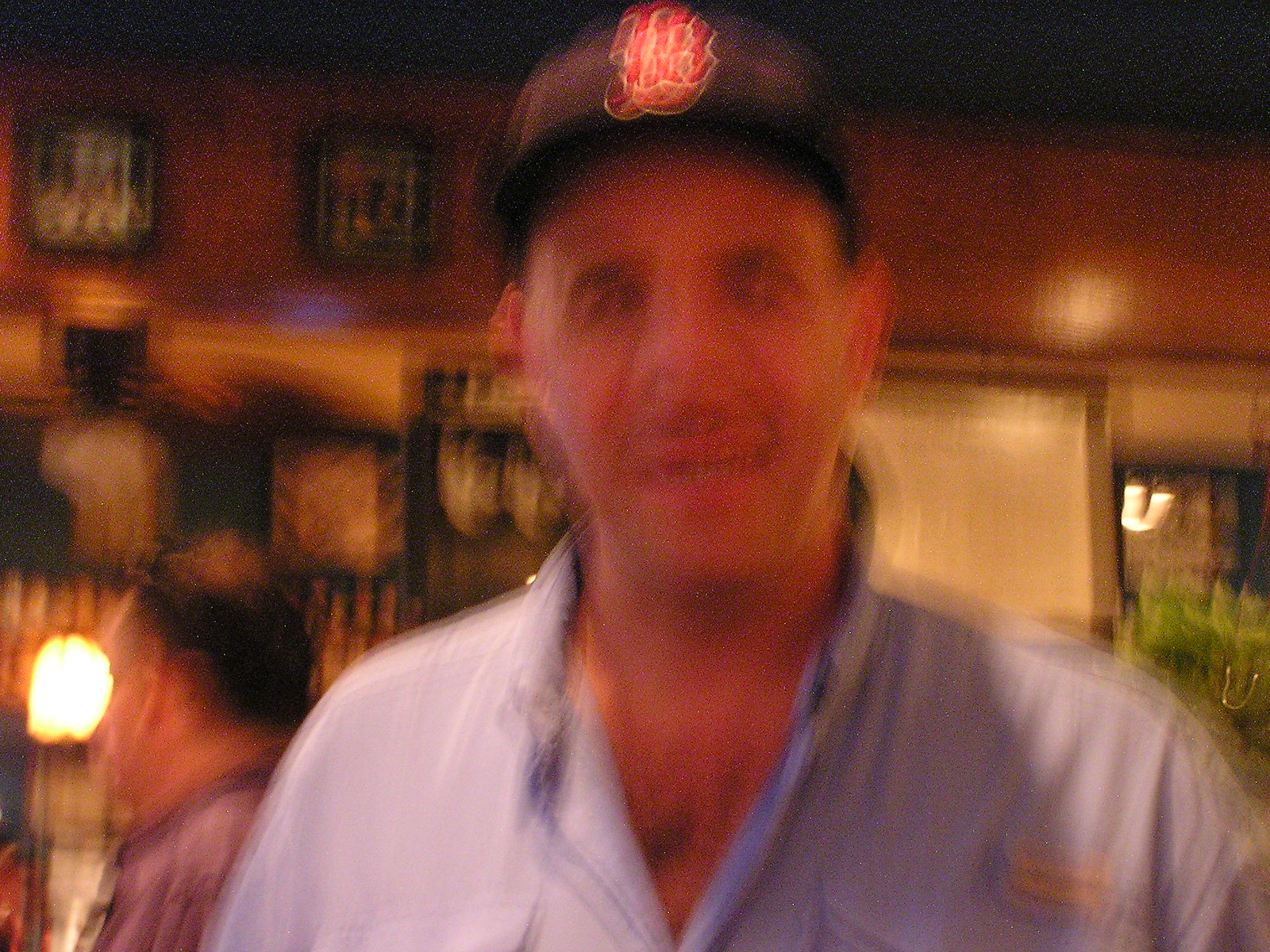The image captures an indoor setting, likely a business establishment such as a restaurant or bar, characterized by a dark brown wooden wall adorned with several framed pictures. The photograph appears very blurry, possibly due to motion or an intentional filter effect, making it difficult to discern fine details. In the lower left-hand corner, a light illuminates part of the scene. The back of a man's head, showing a bald spot and dark hair, is visible; he wears a purple shirt. Dominating the foreground, another man with fair complexion stands directly in front of the camera, wearing a light blue work shirt and a black baseball cap featuring a red symbol, which might be a logo or the letter "B". Behind him, the background includes a mix of potentially green displays, shelves, and a mirror, evoking the crowded and eclectic decor typical of a lively public space.